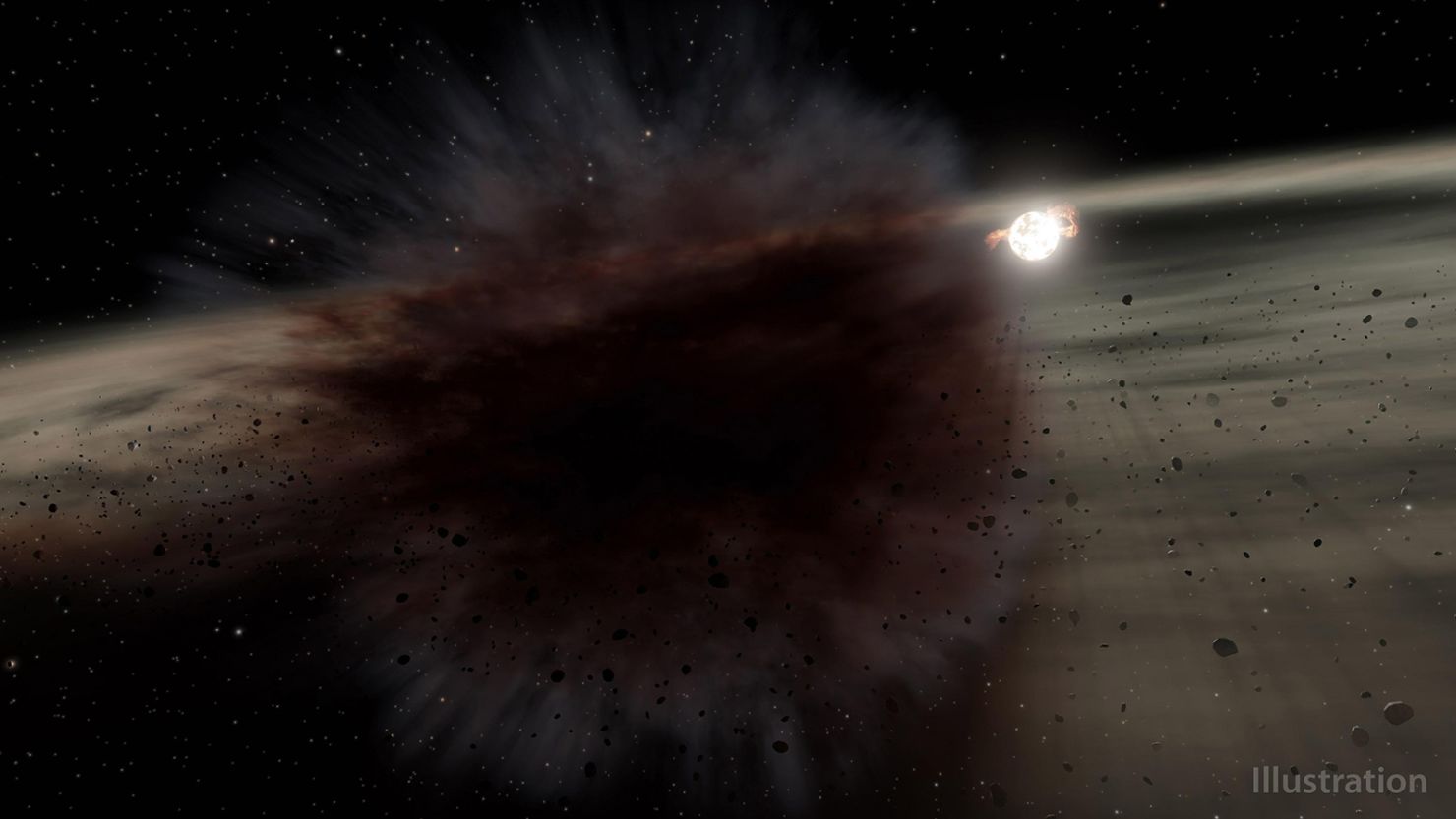The image is a detailed graphic illustration of a cosmic event in outer space. Dominating the scene, the background is pitch black, peppered with countless tiny, bright stars. Stretching across the middle is a grayish-black and white surface, reminiscent of a planet or moon. Central to the image is a dramatic explosion, characterized by a cluster of brown material erupting and releasing a multitude of black particles and gray flames. This explosion seems to create a dust cloud in the immediate vicinity. On the right side, a smaller, incredibly bright white circular object, possibly a star or another celestial body, stands out. This object has a distinctive red line or stripe around its periphery, and its intense light reflects off the surrounding gray debris. The overall scene captures the dynamic and chaotic beauty of a cosmic event, with the detailed interplay between dust, asteroids, and starlight enriching the vast expanse of the universe.